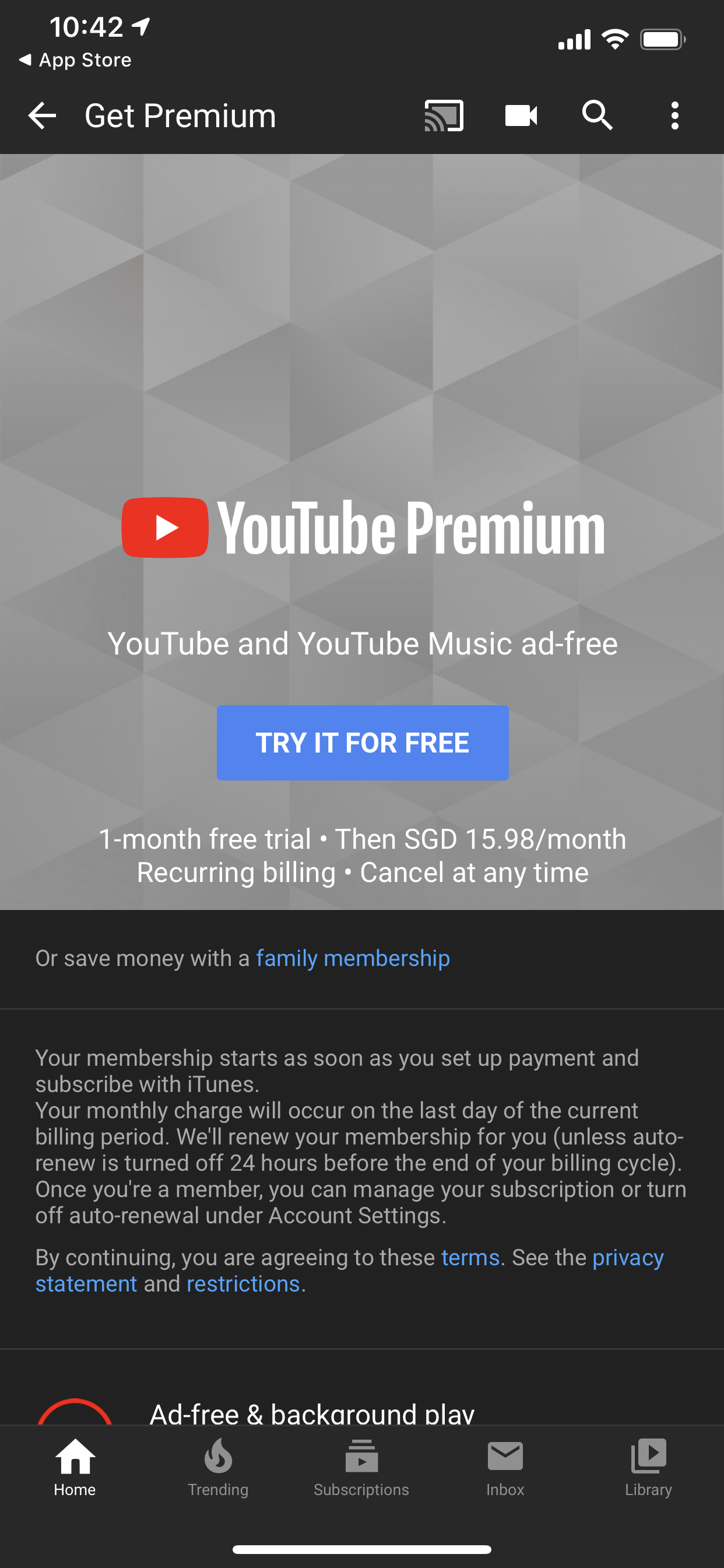This image is a vertical screenshot from a mobile device, showcasing the landing page for YouTube Premium after downloading the app from the App Store. The layout is divided into two horizontal sections. 

The upper section prominently features the YouTube Premium logo and describes the benefits of subscribing, such as ad-free access to both YouTube and YouTube Music. Directly beneath this description is a conspicuous blue button labeled "Try It For Free." Below the button, there is a notification in reversed-out white text on a gray background, informing users about a one-month free trial. Additionally, it mentions the subsequent subscription cost of 15.95 Singapore dollars per month with recurring billing, and the option to cancel at any time.

The bottom section of the screen has a black background with reversed-out gray text. It highlights an additional offer, stating, "You can save money with a family membership." Following this, more detailed information in gray text explains that the membership begins immediately upon setting up the payment. This section includes legal information on the subscription terms, emphasizing the necessity to cancel to avoid future charges.

Overall, this screenshot serves as a promotional display for YouTube Premium, emphasizing its key features and subscription details.